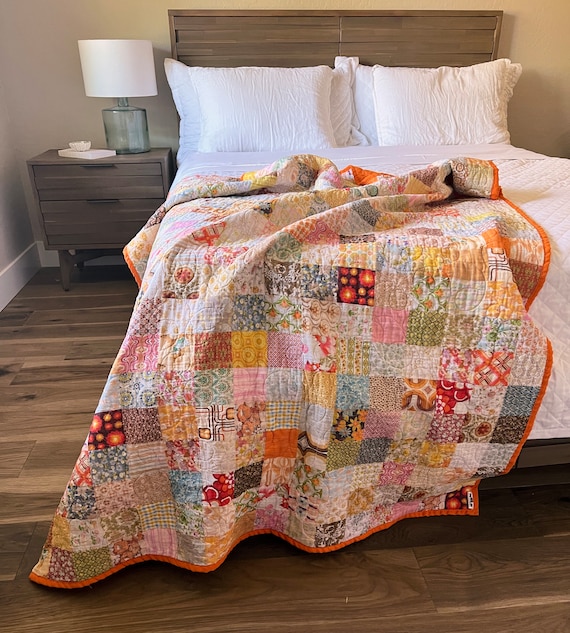This indoor photographic image captures a cozy bedroom with light tan walls and white baseboards. The bed, likely queen-sized, dominates the scene, viewed from the foot of the bed. It features a brown wooden slatted headboard, multiple white pillows arranged up against it, white sheets, and a white quilt. Draped over these is a vibrant, handmade patchwork quilt characterized by its orange trim and diverse, colorful squares with various patterns, including pink florals, geometrics, and circular designs. The quilt is not fully made, with part of it cascading onto the hardwood floor. To the left of the bed stands a matching wooden nightstand with two drawers. Atop the nightstand is a large green glass lamp with a round white shade, accompanied by a plate holding what appears to be an ashtray or bowl. The entire scene exudes warmth and attention to detail, highlighting the inviting and personalized nature of the space.